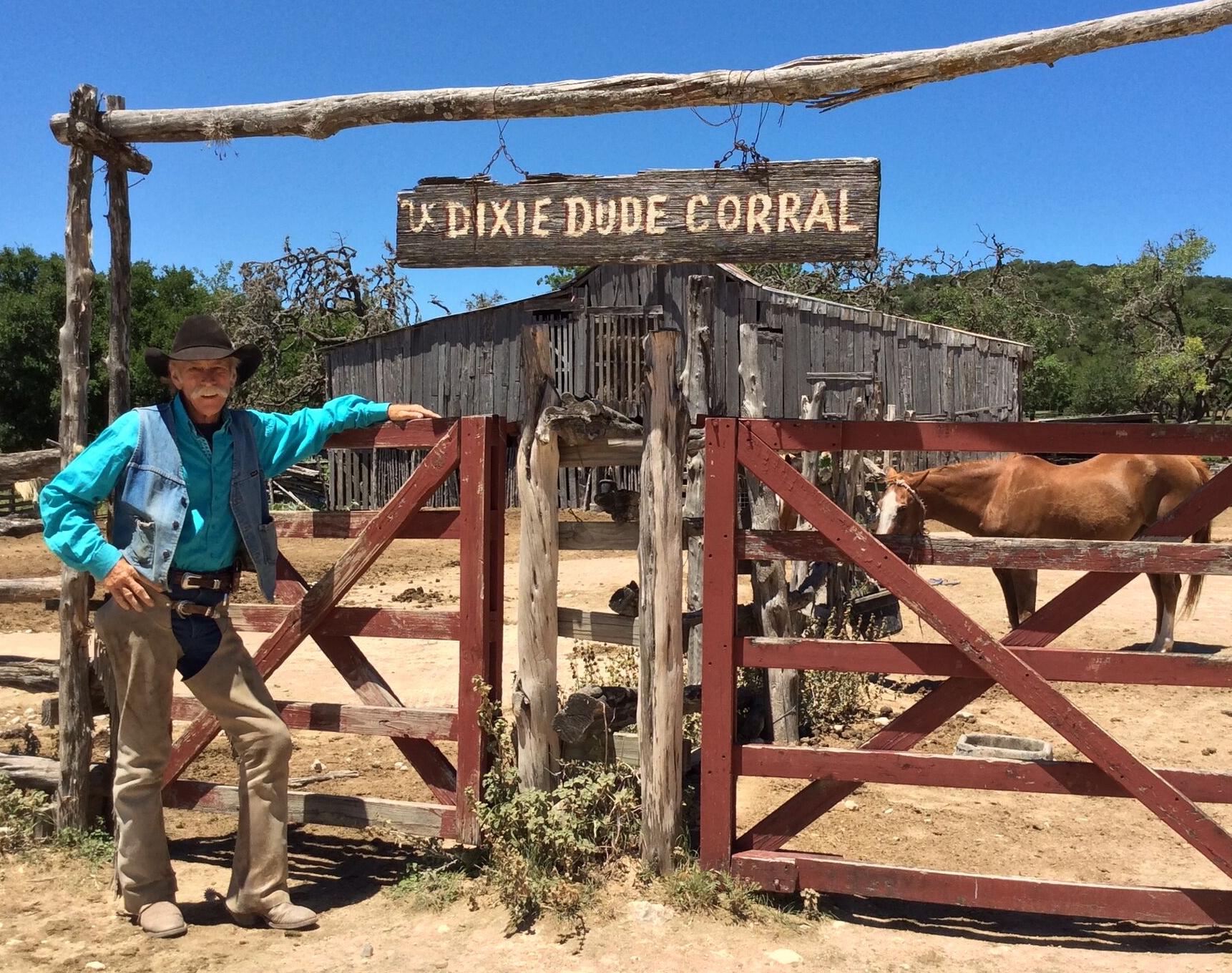The photograph captures a vivid ranch scene bathed in bright sunlight. Set against a backdrop of luscious green hills and a bright blue sky, the rustic charm of the landscape is immediately evident. Central to the image is a weathered wooden ranch gate, painted in a faded red. Natural log fences flank the gate, and a sturdy wooden support structure arches overhead. From this structure, rusted chains dangle a wooden sign carved with white lettering that reads, "Dixie Dude Corral."

On the left side of the gate stands an older, white-haired cowboy. He sports a big white mustache and a dark brown cowboy hat, indented in the front. His attire includes beige leather chaps over blue jeans, shiny belt buckle, and a vivid blue button-up shirt that's brighter than the sky. Over the shirt, he wears a denim vest that hangs open, revealing a black t-shirt underneath. The cowboy, with a grinning smile, leans casually against the gate with a hand resting on it.

To the right of the cowboy and partly hidden behind the right-hand gate, a large chestnut brown horse with a white stripe down its snout gazes directly at the camera. In the background, behind the main gate and fencing, stands a large, dilapidated barn that appears neglected and in need of repair. Green trees and rolling hills stretch out behind the barn, completing the tranquil yet rugged snapshot of this nostalgic western setting.